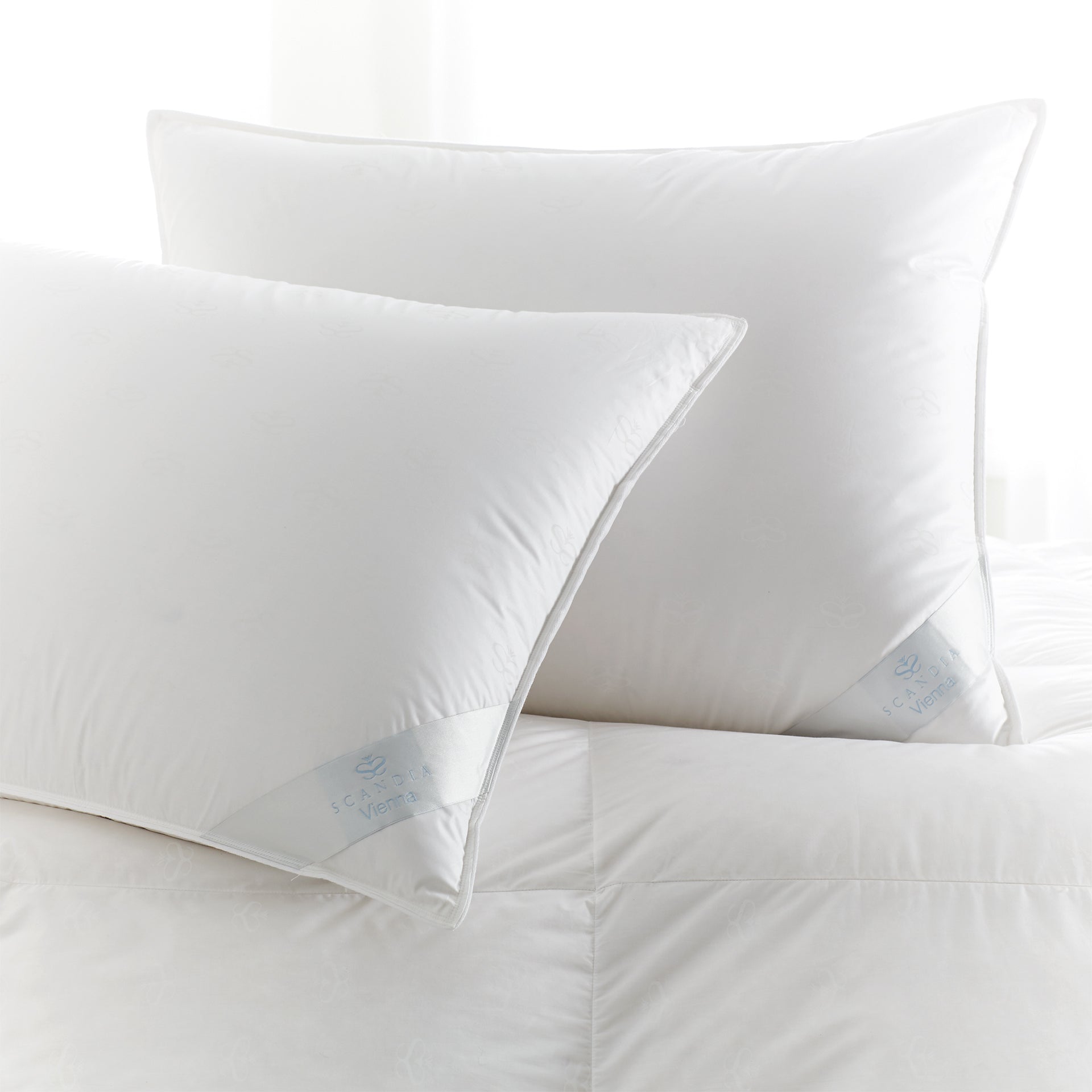In this close-up photograph, two white pillows are prominently displayed, positioned centrally on a white, slightly wrinkled comforter. Each pillow is adorned with a small, silver stripe on their lower right corner, featuring a hard-to-read brand logo in light blue, reflective lettering that likely spells "Vienna." The pillows lack pillowcases, exposing their rectangular shape and stitched edges. A gentle light source from behind illuminates the scene, enhancing the clean and serene atmosphere emphasized by the all-white bedding ensemble.